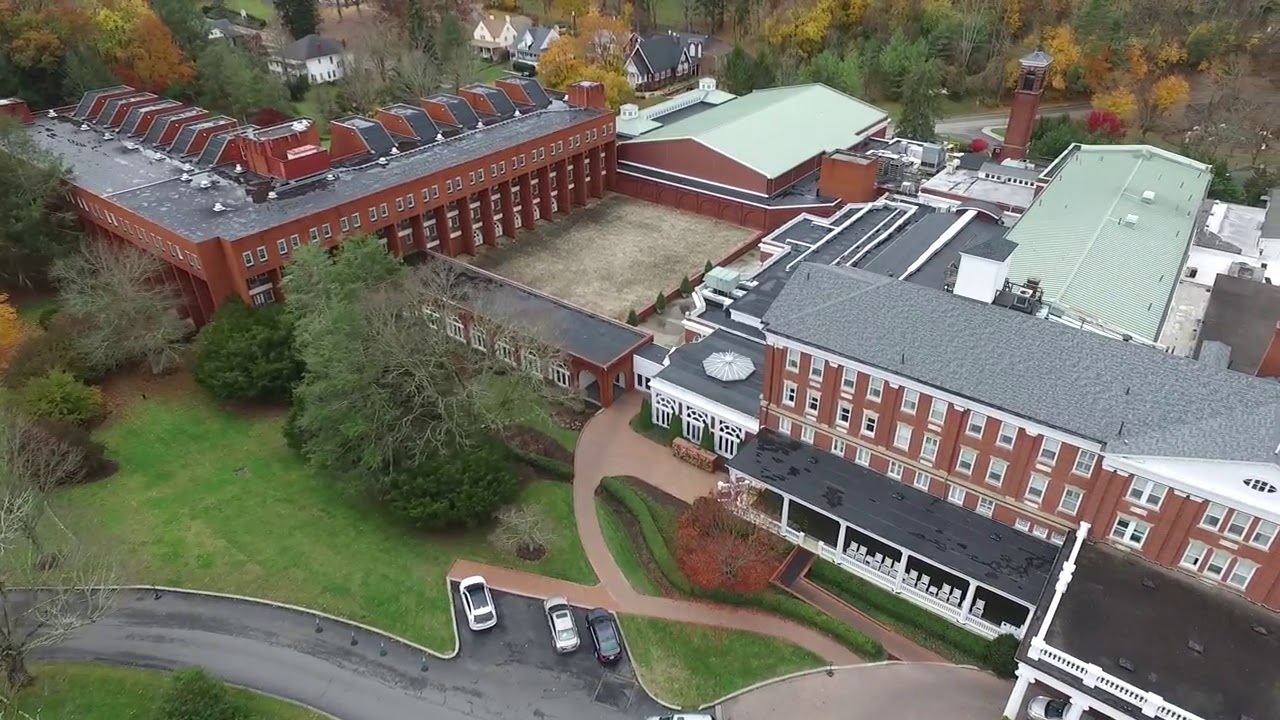This image is a detailed aerial, drone-height color photograph showcasing a sprawling complex of red brick buildings possibly resembling a school or a large apartment complex. The buildings are arranged diagonally from the top left corner to the bottom right. The lower part of the image features a gray paved street with a small parking area where three cars are parked: a white car on the left, another white car in the middle, and a black car on the right. Surrounding the central complex, the roofs predominantly feature gray and black shingles.

In the foreground, to the left of the street, is a green field with scattered trees. Toward the top left, a variety of houses with gray roofs and multiple stories are visible among colorful woods. In the background of the image, there is a prominent large red brick building with a distinctive triangular roof, which could be a gymnasium. This building is connected by a breezeway to another structure, forming a spacious, gray-floored courtyard or plaza between them. A notable feature of the complex is a square red brick bell tower located at the back of the right-hand building.

In the top right corner of the image, additional trees and paved roads can be seen, along with a tower or chimney structure. The photograph is highly detailed and captures the varied architectural elements and natural surroundings, presenting a realistic, comprehensive view of the area.